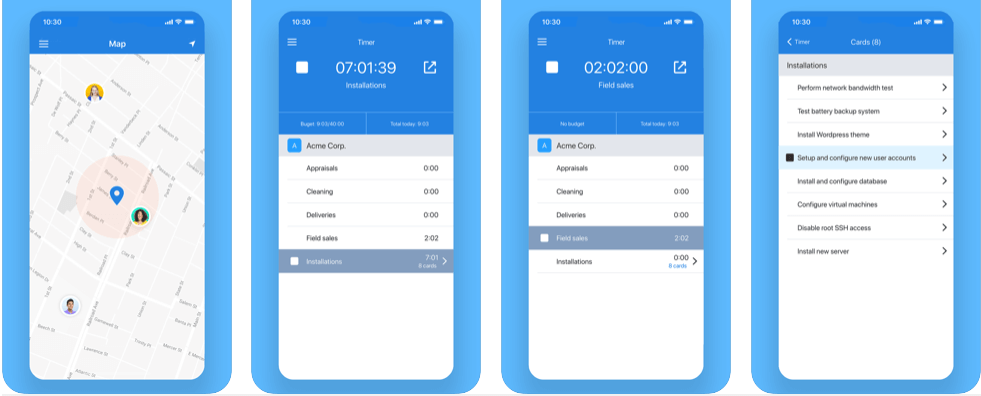Here is a collaboratively refined and detailed caption for the collage of images:

---

This collage features four screenshots captured from a likely iPhone, all set against a light blue background. 

1. The first image showcases a map interface with a light grey map background displaying street names. Three small icons, each representing different people, are positioned around the map. A blue pin marks a specific location at the center. Above the map, a blue bar with the word "Map" in white is visible, flanked by a location icon on the right and a drop-down menu option on the left.

2. The second image highlights a timer interface displaying "7 hours, 1 minute, and 39 seconds". To the left of this timer is a "Stop" button, and to the right is a "Share" button. Below the timer, the word "Installations" is visible, followed by a list of options: "Acme Corp", "Appraisals 0", "Cleaning 0", "Delivery 0", and "Field Sales 202". There's also a greyed-out option labeled "Installations 701".

3. The third screenshot also displays a timer, this one showing "2 hours, 2 minutes". Beneath the timer is the label "Field Sales," which correlates with the list of options below the timer in the same format as the previous image, where "Field Sales" is highlighted in grey.

4. The fourth screenshot is titled "Cards (8)" and appears to list tasks under the heading "Installations". The tasks are: 
   - Perform network bandwidth test
   - Test battery backup system
   - Install WordPress theme
   - Setup and configure new user accounts
   - Install and configure database
   - Configure virtual machines
   - Disable root SSH access
   - Install new server

---

This caption provides a comprehensive and detailed description of the images in the collage.